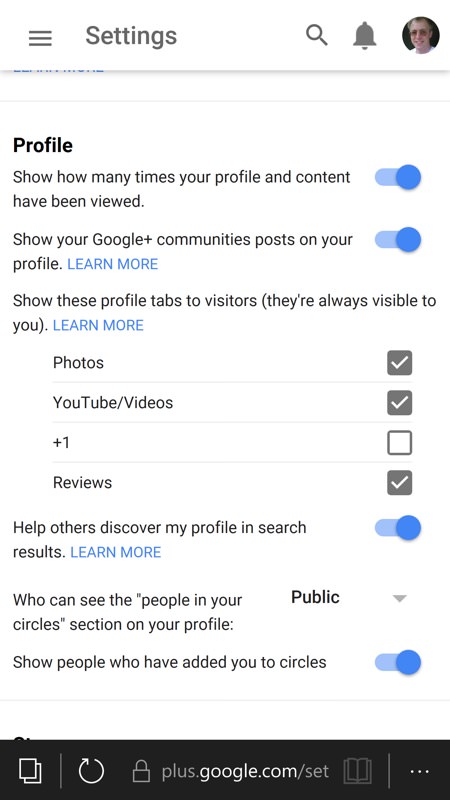Detailed Caption for Screenshot:

The screenshot captures the settings menu of a legacy Google+ profile. The screenshot appears to have been taken on a mobile device. At the top right corner of the interface, there's a user profile picture adjacent to a notification bell and a search icon, indicating the user is logged in.

In this settings menu, the first visible option is to show how many times the user's profile and content have been viewed, which is toggled on. Directly below that, there's an option for displaying Google+ community posts on the user's profile, which is also activated.

The menu includes multiple instances of “Learn more” links in blue text, designed to provide additional information about the settings. The section titled “Show these profile tabs to visitors” lists several checkboxes, all marked as checked:
- Photos
- YouTube videos
- +1s
- Reviews

Each of these categories will be visible to profile visitors. There's another setting labeled "Help others discover my profile in search results," which is toggled on, accompanied by a “Learn more” link.

Further down, the settings specify who can see the people in the user’s circles, which is set to public. Another setting indicates that showing people who have added the user to their circles is activated.

At the bottom of the screen, there’s the URL "plus.google.com/set," a refresh button, and a tab button, all on a small, black bar. On the right-hand side, there’s a contact meeting icon.

This detailed setup shows various privacy and visibility options tailored for a Google+ profile, reflecting the personalization efforts available on the now-defunct social media platform.